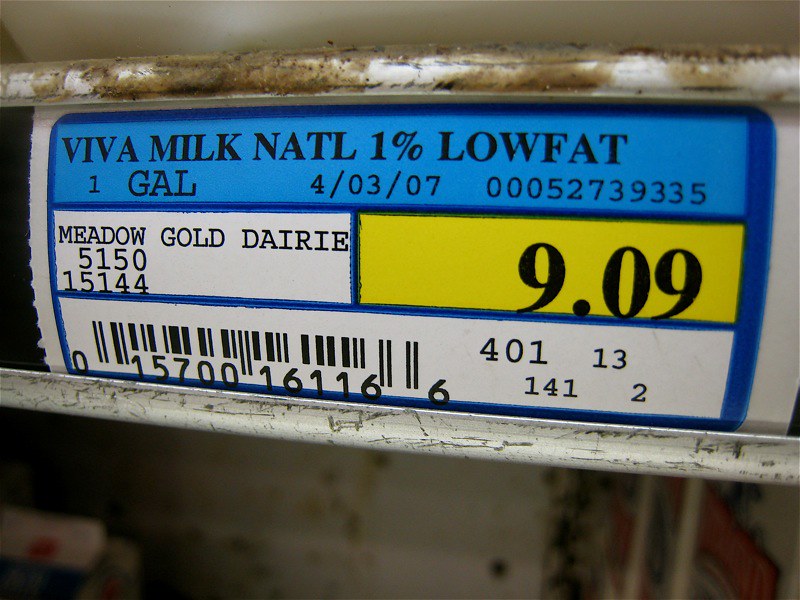This close-up photograph features a food item label displayed on the front of a supermarket shelf. The metal components of the shelf, positioned above and below the label, show significant signs of wear and tear. The once-white paint has chipped away, revealing the underlying silver metal, particularly on the bottom section. The top part of the shelf appears quite dirty, with brown, dried smears, possibly from food or dirty water, indicating neglect.

The label itself is clean and rectangular, stretching from the left to the right edge of the image. It is divided into three horizontal sections, each separated by a blue border. The top section features a dark blue border and a lighter blue background. Here, the text in black reads "Viva Milk NATL," followed by "one percent low fat," and "one gal." Below this, a date is listed: "04/03/07," beside a number: "0005273935."

The middle section is split into two halves by a vertical blue line. On the left half, black text on a white background reads "Meadow Gold Dairy 5150," with "15144" underneath. On the right half, a bold black "9.09" is prominently displayed on a yellow background.

The bottom section features a barcode starting from the left side, whose numbers read: "015700 16116 401 13 141 2."